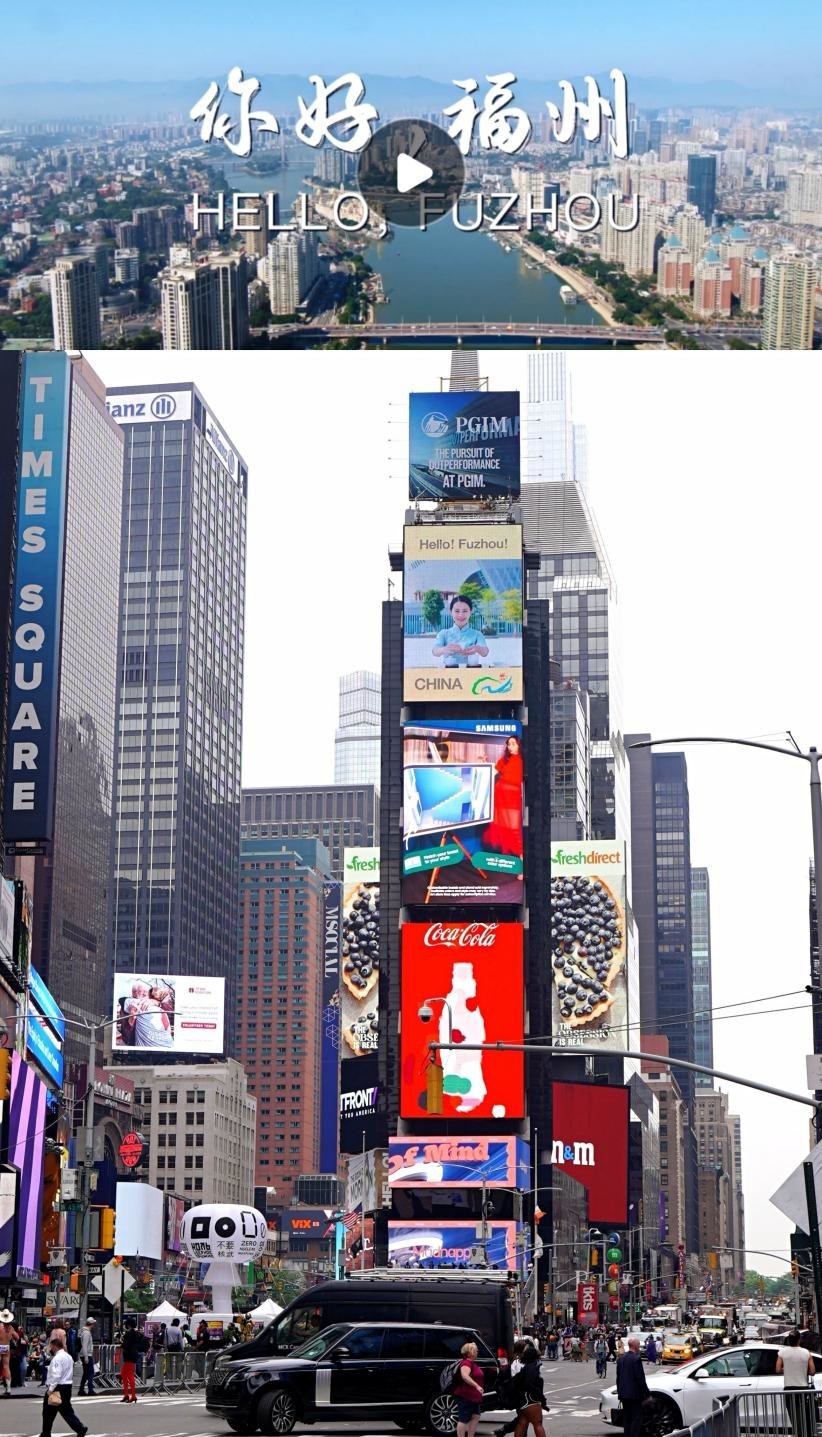The image is divided into two sections. The top one-sixth of the image features a screenshot of a video, identifiable by a play button overlaid in the center. This video shows a city skyline with a canal running through it, set against a backdrop of barely visible mountains shrouded in fog. The sky is a clear blue. There are two lines of text in the center of this top section: the upper line is in Chinese characters, and the lower line, in bold capitalized white letters, reads "HELLO, FUZHOU."

The bottom portion of the image depicts a bustling city square reminiscent of Times Square. Dominating the scene are numerous vertically tall digital billboards displaying various advertisements, including a prominent Coca-Cola ad. The square is filled with cars—a black SUV, a black van, and a small white vehicle—while crowds of people traverse the streets, suggesting an event is underway, evidenced by guardrails set up to manage the pedestrian flow. The atmosphere is energetic with the busy streets and vibrant ads, encapsulating the essence of a lively urban environment.